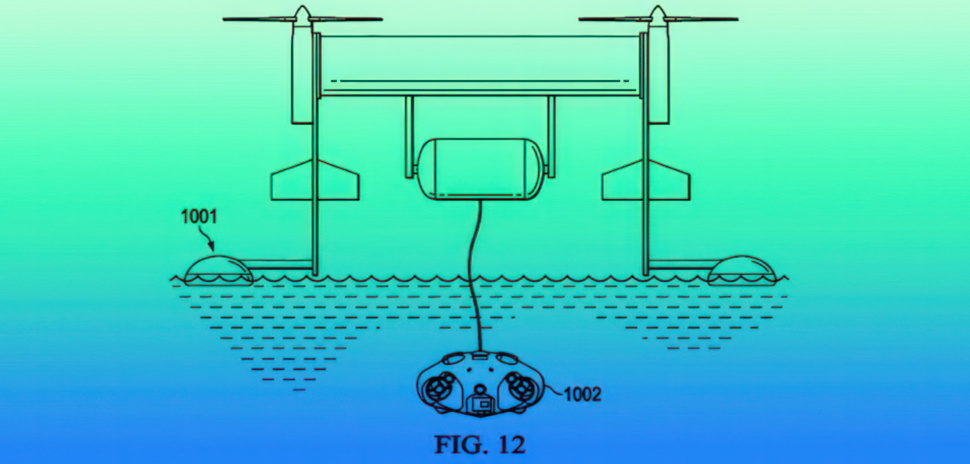The rectangular image, measuring approximately five to six inches wide and three inches high, transitions from a blue background at the bottom to green and then light mint green towards the top. In the bottom center, black text reads "FIG. 12." The main focus is a detailed schematic drawing, indicating a device that interacts with both air and water. 

At the center of the image, floating above the water, is a main structure with a square-like appearance. On the top left and right corners of this structure are propellers. Just under this structure, labeled as "1001," are buoy stabilizers, suggesting the device's capability to stay afloat. A cable extends from this structure, connecting to an oval-shaped submersible object beneath the water, which appears to be an underwater apparatus. This sub is labeled "1002" and resembles a remote control handle with thumb wheels or joysticks on either side, possibly indicating controls or propulsion mechanisms.

The submersible is tethered by a single black line, likely a hose or cable, which indicates it is connected and possibly dependent on the main floating structure. Surrounding this setup, there are subtle wave illustrations that emphasize the aquatic nature of the device. The combination of the propellers and submersible hints at a multifunctional system designed for both aerial stability and underwater exploration.